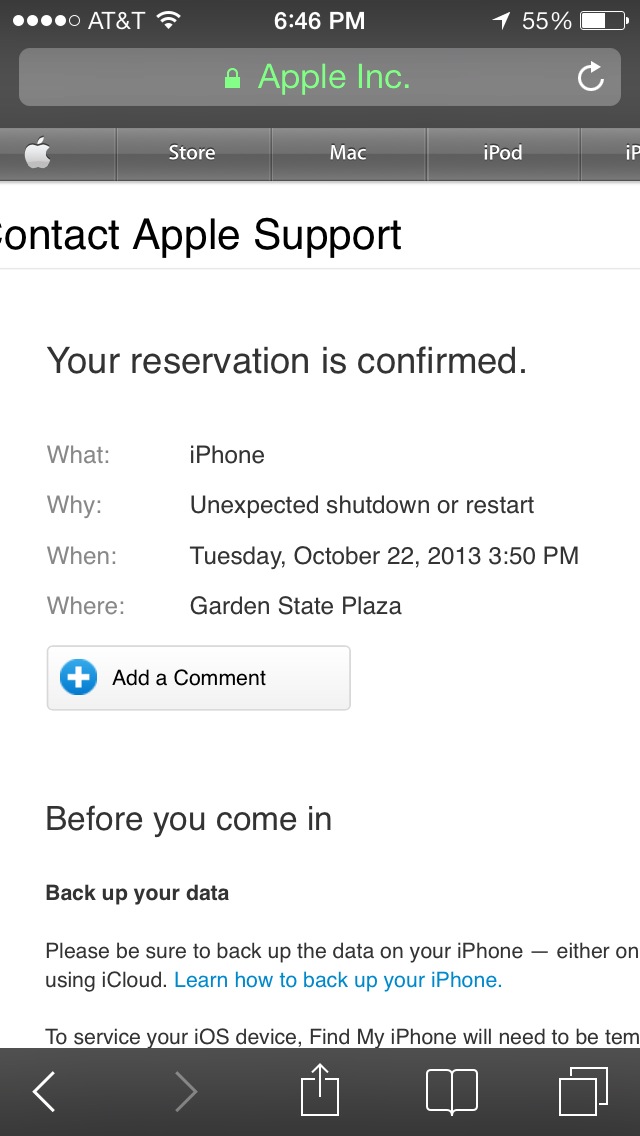This image is a color screenshot taken from an Apple iPhone in portrait orientation, displaying a reservation confirmation for Apple support in the Safari browser. The top bar is dark, featuring various device statistics such as the time (6:46 p.m.), signal strength, Wi-Fi connection, GPS status, and battery percentage. The address bar reads "Apple Inc." with a lock symbol beside it, indicating a secure connection. Below this, an older Apple navigation bar appears, showcasing small icons and links to sections like the Apple Store, Mac, and iPod.

In the main section of the screenshot, the title "Contact Apple Support" is prominently displayed, followed by the confirmation message "Your reservation is confirmed." Detailed information about the reservation includes:
- **What:** iPhone
- **Why:** Unexpected shutdown or restart
- **When:** Tuesday, October 22nd, 2013, 3:50 p.m.
- **Where:** Garden State Plaza

A button labeled "Add a comment" is shown beneath this section, accompanied by a blue circle with a white plus sign. Further instructions advise the user to back up their data before the appointment, providing a link to learn how to back up using iCloud. The bottom of the screenshot features navigational icons typical of a Safari browser, including the back, forward, share, bookmark, and tab buttons.